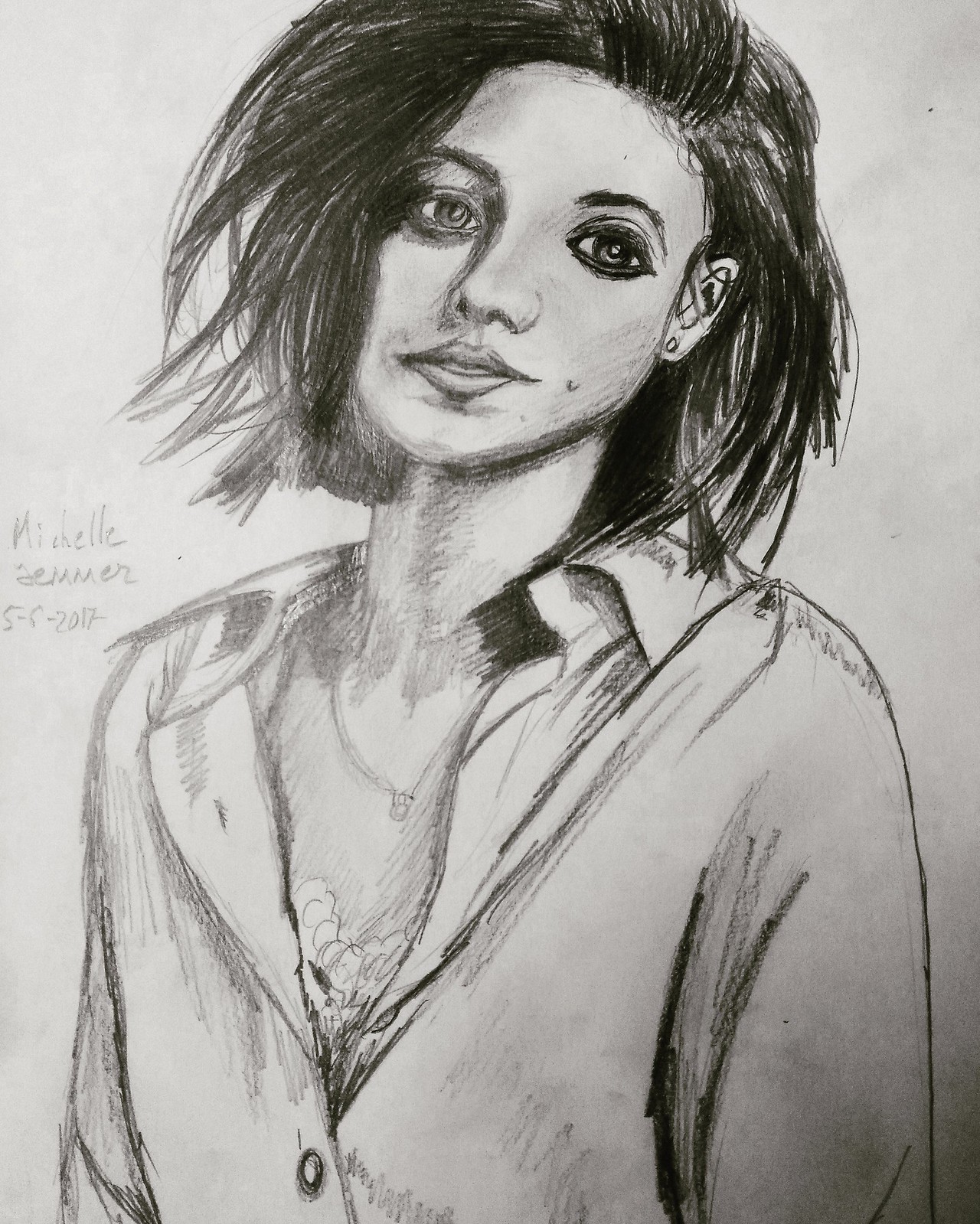The image is a detailed black and white sketch of a woman named Michelle Semmer, dated 5-5-2017. The drawing captures a realistic portrayal of a female with long, silky black hair, slightly tilted to the right. She has a mole on her left cheek. Her eyes are distinct, with the left one shaded darker than the right, giving her a unique expression. A subtle smirk reveals the top of her teeth. Michelle is adorned with a grey necklace featuring a circular pendant, and an earring is visible on her left ear, which appears on the right side of the image. She wears a collared coat, buttoned at the bottom, over what seems like another layer of clothing beneath. The background remains white, accentuating the sketch's details, and her name, "Michelle Semmer," along with the number "5527," is written on the left side of the artwork.